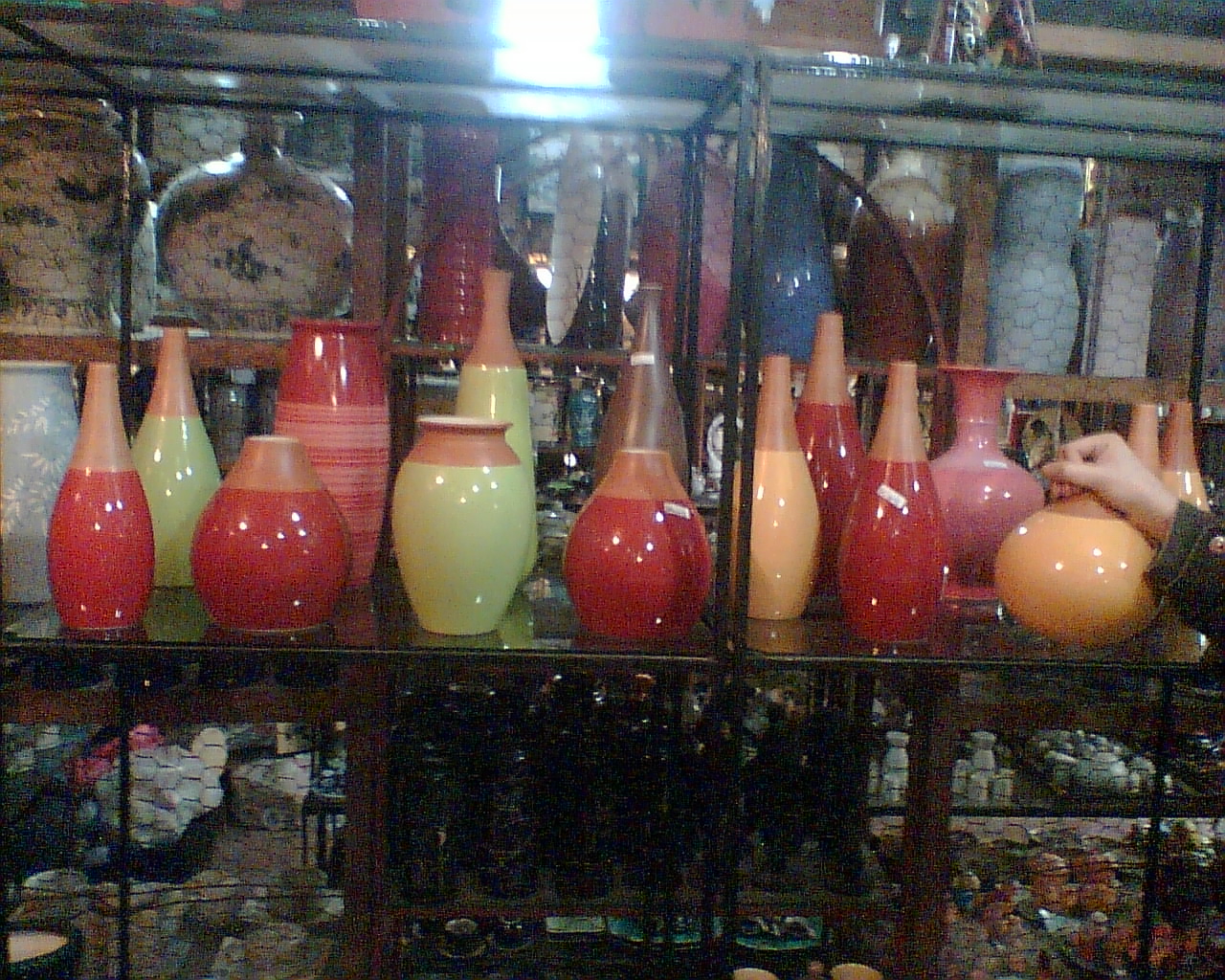The image depicts a detailed scene in a pottery store featuring an array of vases displayed on a series of black wooden shelves. The top shelf has glass on it, showcasing several vases and pottery items that are partly visible. Each vase appears meticulously crafted, with many sharing similar shapes, such as those resembling champagne or wine bottles, while others have broader bottoms tapering to narrower necks. The glazing on the vases is predominantly a peachy color, burnt red, pale green, and often creates a striking two-toned effect, typically tan combined with another color. Also notable is one blue-gray vase with a white design work on the left side. 

The middle shelf prominently displays a variety of vases, highlighted by the bright lighting from the center top of the frame. One of the middle vases, a pink one with a bulbous bottom and smaller head, is being reached for by a woman’s right hand, identifiable by its painted nails and the cuff visible on her sleeve. Further in the background, other shelves hold larger pottery pieces and smaller miscellaneous items, many obscured by a protective black chicken wire. Below the vases on the main shelf, smaller knickknacks create a busy backdrop. Overall, the scene is rich with terracotta tones and glazed finishes, evoking a warm, artisanal ambiance.